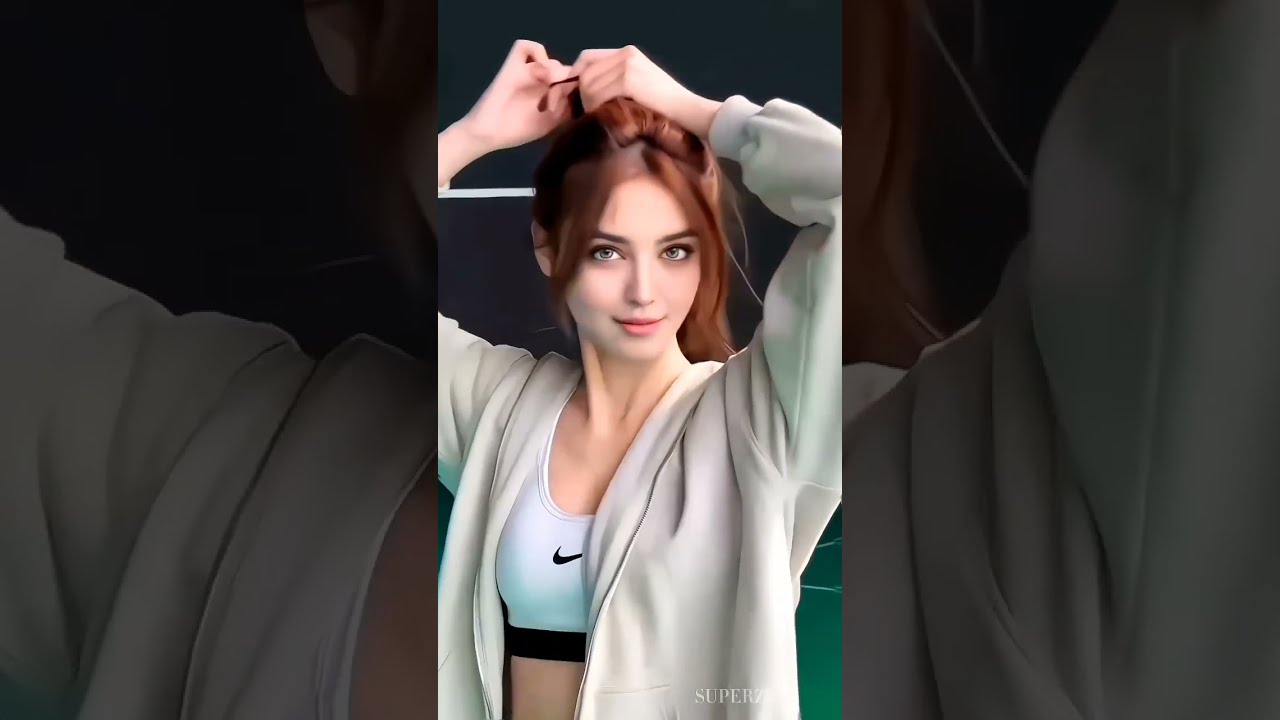The image features a young woman with red hair styled in curtain bangs, who is arranging her hair into a high ponytail. Her fair skin accents her striking features as she looks straight ahead, smiling with her mouth closed. She is adorned in a gray-green zip-up hoodie jacket, left open to reveal a white Nike athletic top underneath, distinguished by a black swoosh logo and a black band at the bottom. Her hands are positioned above her head as she ties her hair, adding a dynamic element to the portrait. The photograph is vertically cropped, emphasizing her from the waist up, with two black bars framing the inner, middle center of the image, possibly accentuating the photo's central focus. The woman appears to be standing on a green surface with white stripes, reminiscent of a tennis court, set against a contrasting white and black background.